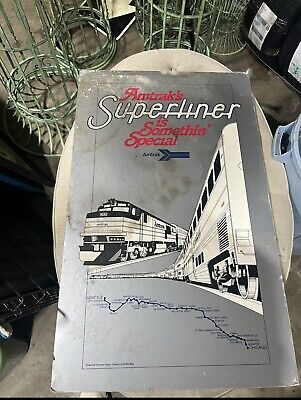The photograph depicts a vintage Amtrak Super Liner flyer, predominantly metallic silver in color. The flyer features the phrase "Amtrak's Super Liner" in bold white text outlined in black, followed by "Is Something Special" in red italicized font. Below this text, there is a detailed black-and-white illustration of the Super Liner train, showcasing the front of the train and a side view, with a map-like line indicating its route. The flyer is placed on top of a beige seat cushion in what appears to be a cluttered room. The background is filled with several wire baskets, the bases of metal tables, and a bucket positioned towards the right side, adding to the disarray. The chair, an oval-shaped white leather stool without a back, supports the nostalgic advertisement amid the surrounding clutter.